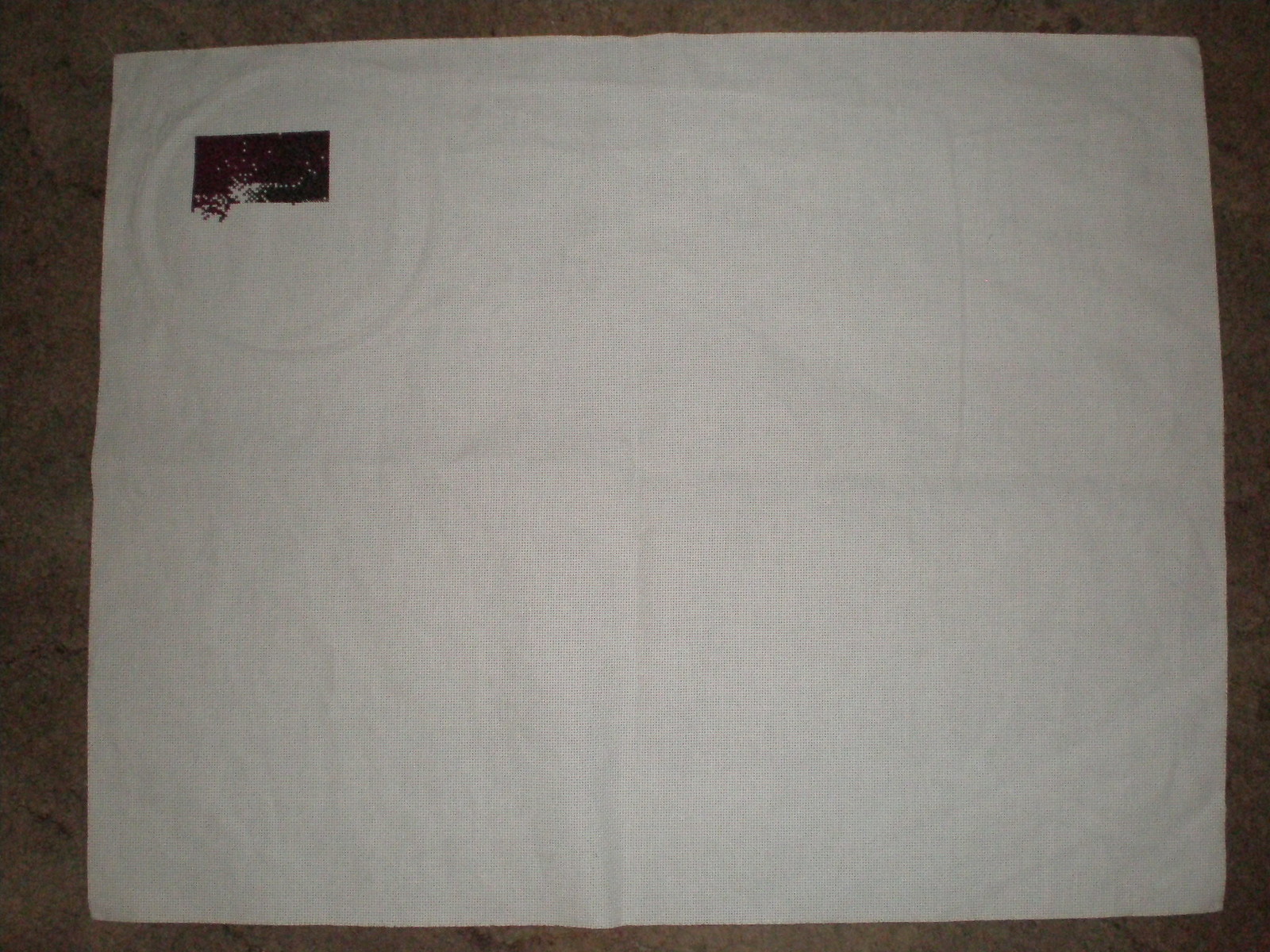On a dark brown background, a pristine white cloth, nearly covering the entire surface of the table it rests on, takes center stage. In the upper left-hand corner of the scene, an intriguing black mark draws the eye. This mark, not quite square and more oblong in shape, appears to depict a tiny segment of a night sky. Scattered within this dark patch are minute, star-like specks, culminating in what resembles a small cosmic explosion. The white cloth itself bears evidence of prior use, featuring a rounded impression as if a large, circular object had recently rested upon it. Accompanying this indentation are numerous wrinkles, adding texture and depth to the scene.